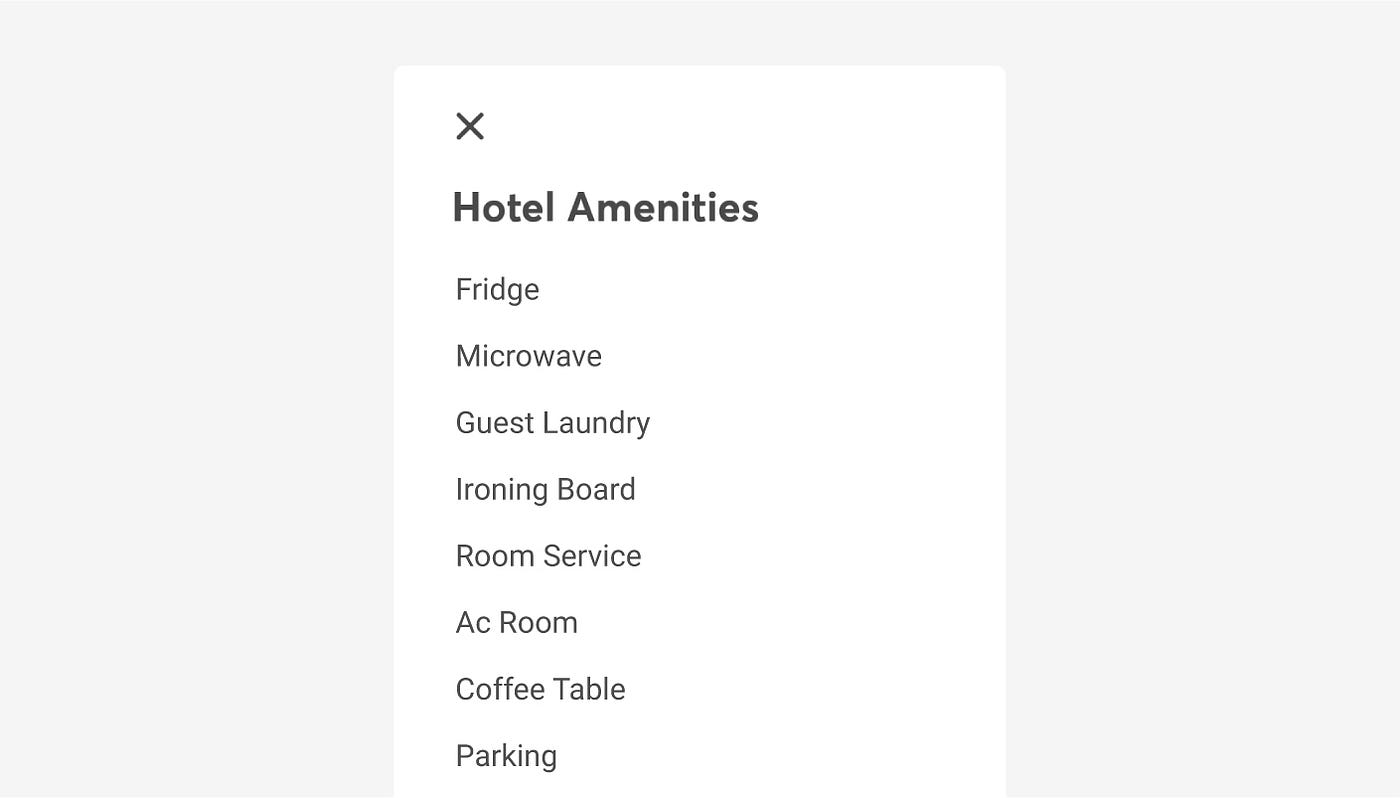The image features a rectangular composition with a light grayish background. Centered predominantly in the image is a larger white rectangle, extending from slightly below the top margin and appearing to possibly continue beyond the bottom edge. In the top left corner of the white rectangle, there is a black 'X' icon, reminiscent of a window close button. Below the 'X', the phrase "Hotel Amenities" is prominently displayed in bold black text. 

Beneath the header, a list of hotel amenities is provided in smaller, non-bold black text. The amenities include:
- Fridge
- Microwave
- Guest Laundry
- Ironing Board
- Room Service
- AC Room (indicating air-conditioned rooms)
- Coffee Table
- Parking